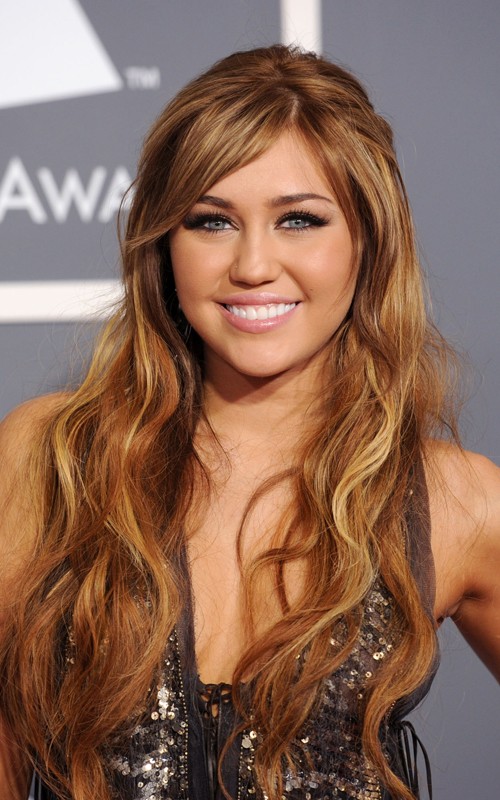This is a tall rectangular photograph of a young woman smiling brilliantly into the camera, captured from the chest up. She has tan white skin and beautiful, very long, curly, blonde-reddish, honey-colored hair that cascades down to her chest, with bangs swooping to the left. Her light blue-gray eyes stand out, enhanced by thick black eyeliner and mascara, framed by light brown eyebrows. She’s wearing light pink lip gloss, and her smile reveals the top row of her teeth. The woman is dressed in a brown sequined top with a very deep V neckline, which laces up the front, showing her bare shoulders and one arm slightly poking out. The top's front glimmers with silver scales-like details. The backdrop is a gray wall adorned with a somewhat blurred logo that includes white capital letters, partly reading "AWA".